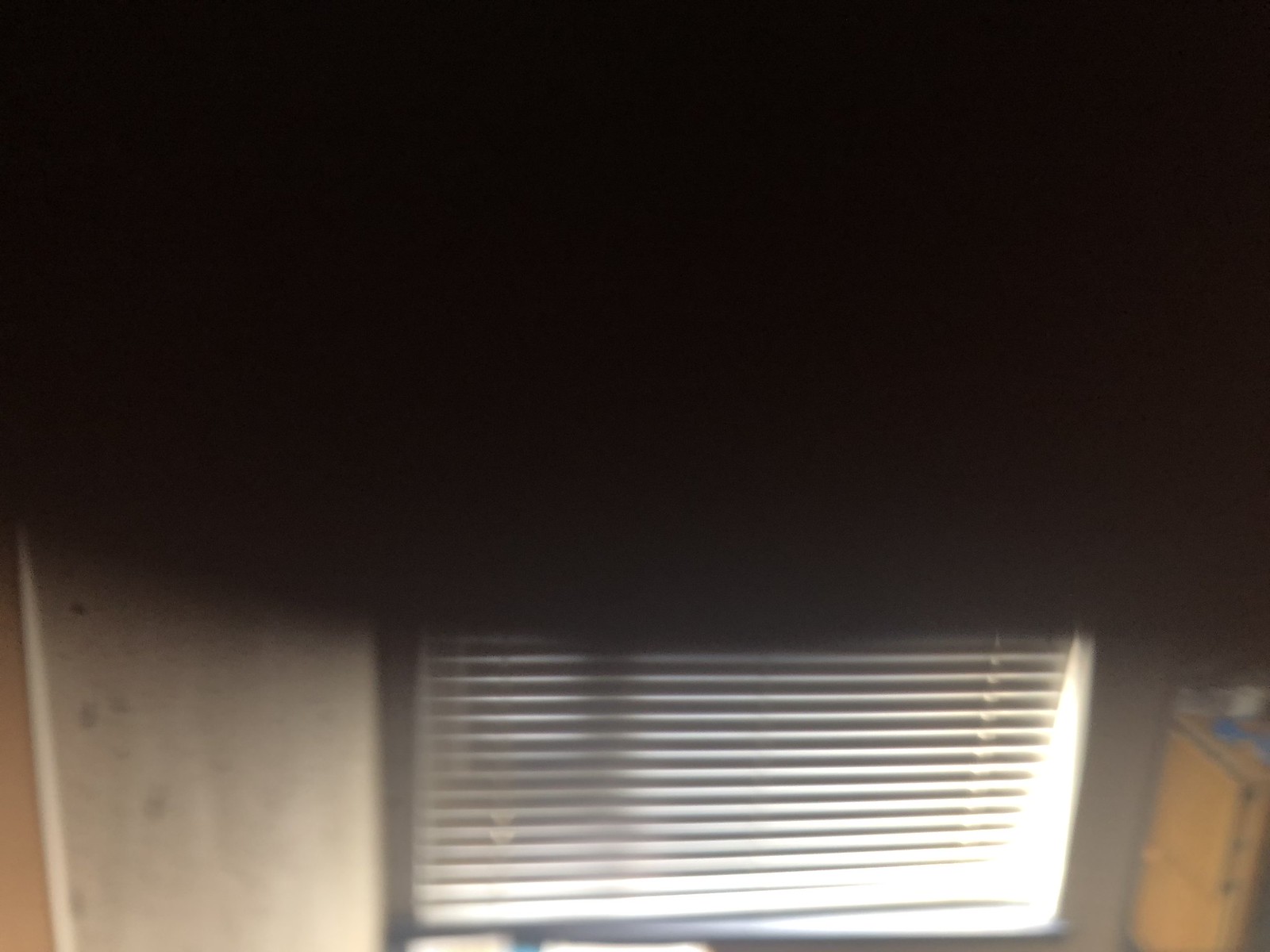The photograph appears to be taken indoors and shows a dark scene with the upper portion almost entirely black, suggesting either a camera malfunction or an obstruction like a finger covering the viewfinder. The lower part of the image starts to lighten up, revealing more details. On the left side, there's a tan wall speckled with black, while the same wall color extends to the right. In the center, there's a window with white mini blinds slightly ajar, allowing a sliver of sunlight to shine through and cast shadows to the right. The window sill is white. On the right side of the photo, there's a light brown desk or possibly a chest of drawers, though the image is too grainy to confirm specific details. The blinds and the sunlight create vertical white lines against the darker backdrop, adding a contrast to the scene.